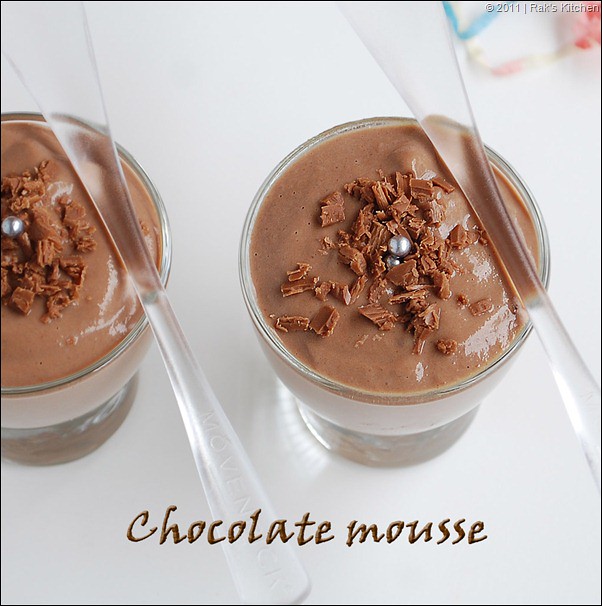The image showcases two small, clear glass cups filled to the brim with rich, chocolate mousse. From a nearly bird's-eye view, we see that the mousses are generously topped with brown chocolate shavings and adorned with round, silver edible pearls. Resting on the top right of each cup is a sheer, transparent spoon, likely made of plastic, which complements the desserts' elegant presentation. The background is stark white, highlighting the decadent brown mousse and the decorative toppings. At the bottom edge of the image, brown text reads "chocolate mousse," tying together the visual and textual elements of the scene.